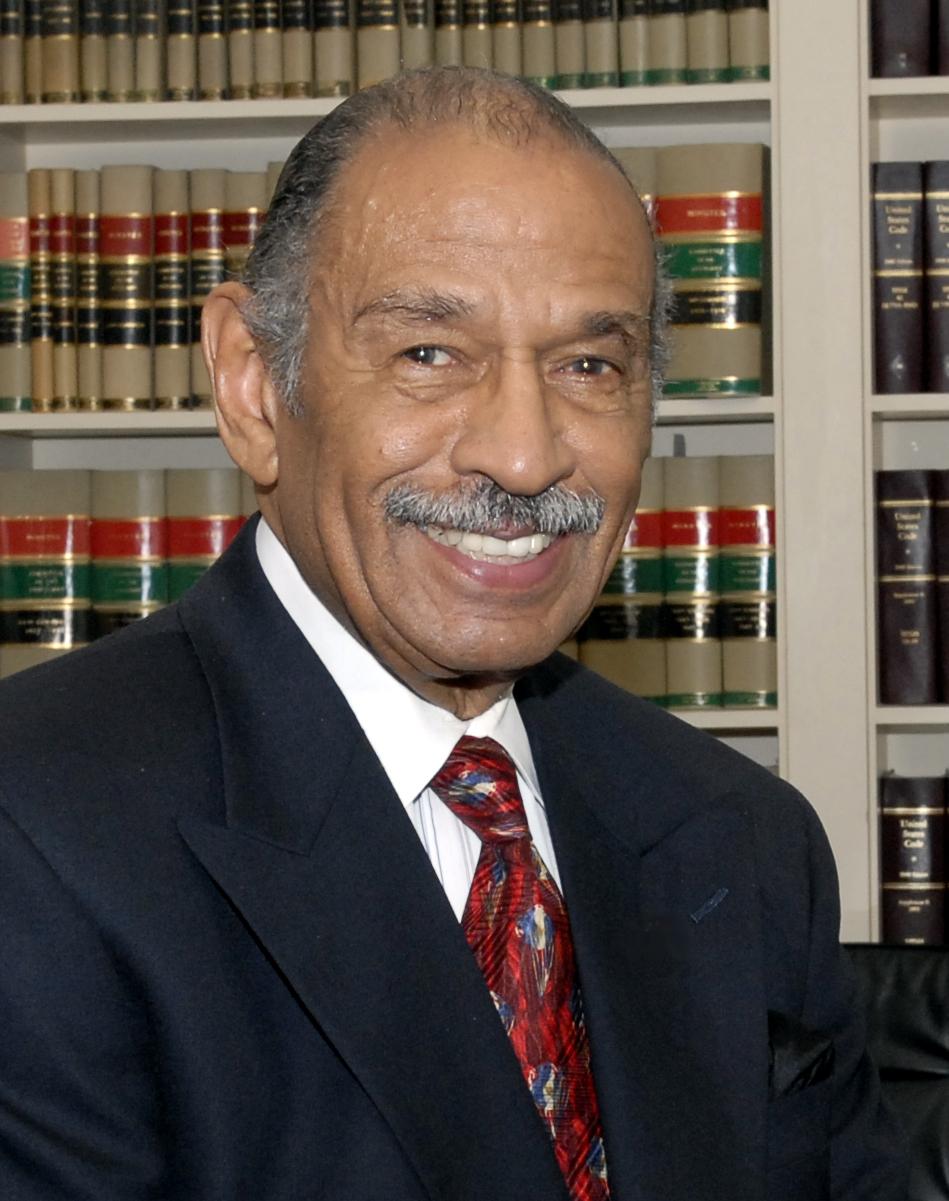The photograph captures an older man with brown skin, a receding hairline, and predominantly gray hair, complemented by a gray and black mustache. His mustache, mostly gray on the outer sides and black at the center, frames his big wide smile, revealing his shiny teeth. He is dressed in a black suit, a white collared shirt, and a red tie featuring dark and light red stripes interspersed with jellyfish patterns. His body is angled diagonally to the right, with his face turned directly towards the camera, light softly illuminating his features.

Behind him is a large white bookshelf filled with volumes of books. The books on the left side are cream-colored with red, green, and black labels. A vertical divider creates a visual boundary, separating these from another section on the right, which contains some black leather-bound books. The man's image is framed from his chest upwards, positioning him in the foreground against this academic backdrop.